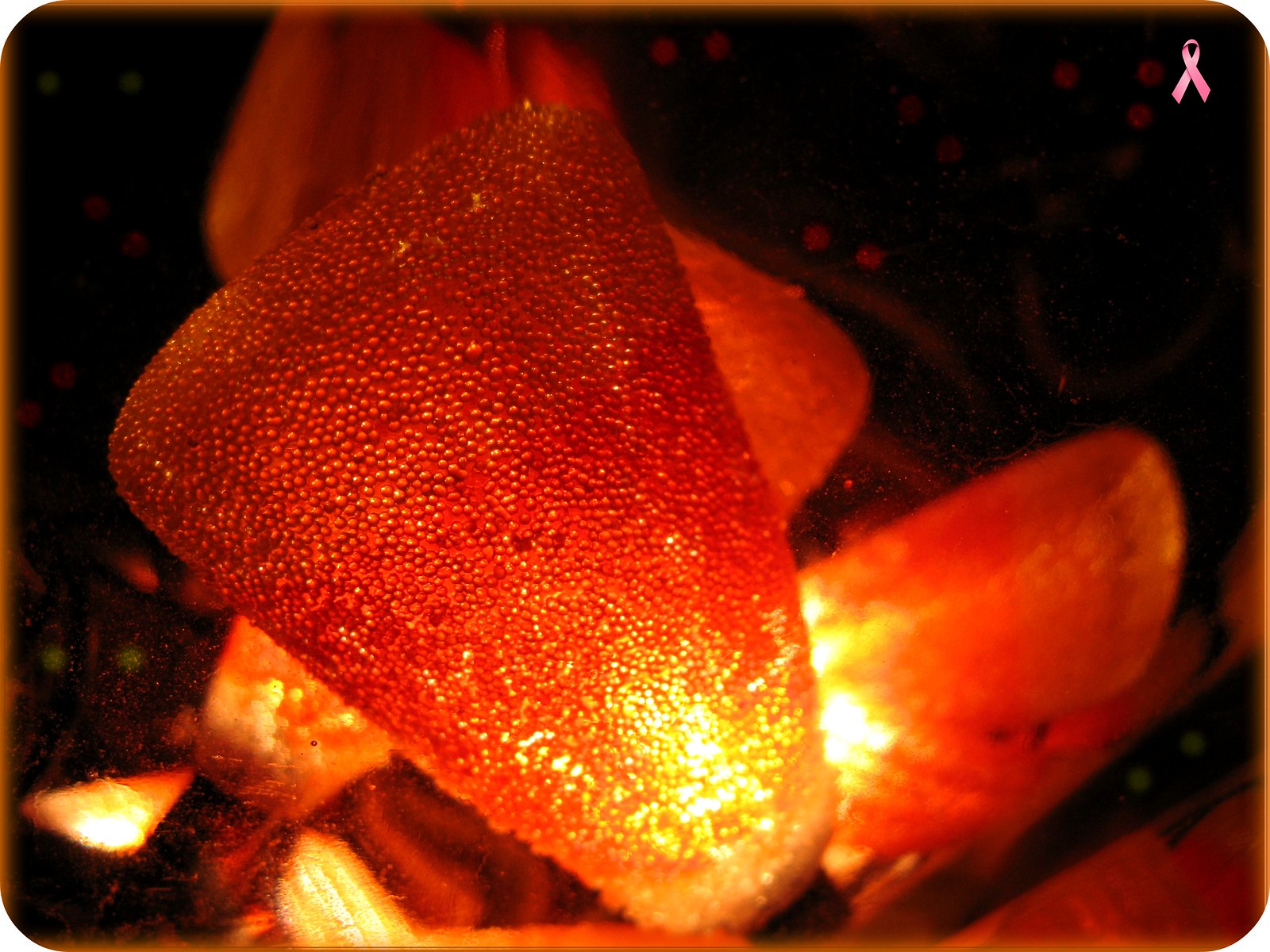The photographic image, set indoors, features a dynamic, fiery scene at its core. Dominating the center, a triangular object, resembling heated iron, displays a gradient from bright red to a glowing yellow at its thinnest point. This object, with tiny bead-like dots reminiscent of an upside-down thimble or even a piece of candy corn, evokes a sense of intense heat as if it's burning from within. Behind this triangular element is an orange, tear-shaped object, also glowing with yellow hues, resembling the curved back of a boat. Another similar orange and yellow triangular element is visible in the background, contributing to the fiery ambiance. In the upper right corner, a pink ribbon symbolizing breast cancer awareness stands out against the heated backdrop. The image is striking with its vivid contrast between the fiery elements and the symbolic ribbon, drawing attention to both the intense heat and the significance of the ribbon.